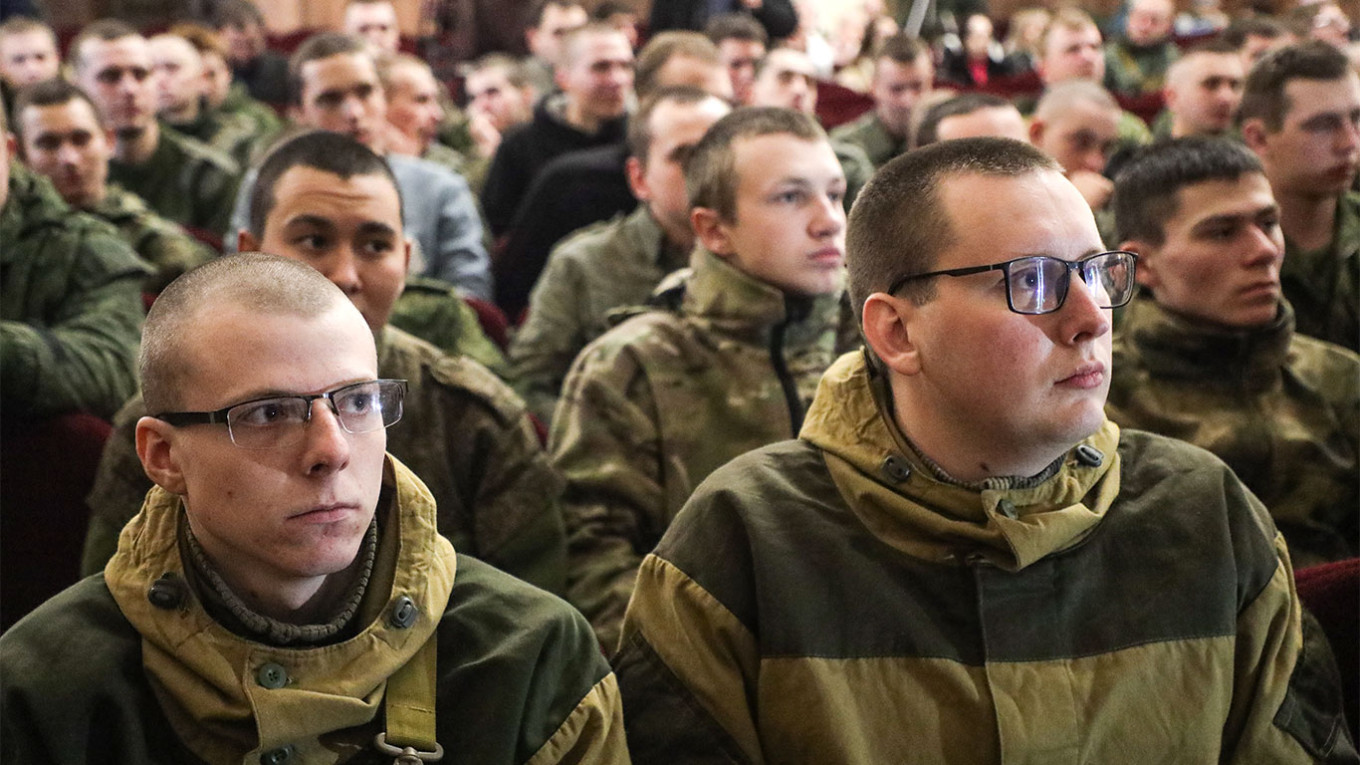The image shows a group of around 50 young men or boys, possibly of Eastern European descent, standing together in what appears to be an auditorium. The majority are dressed in military-style apparel, including camouflage jackets, while others wear uniforms with a distinctive striped pattern featuring dark green around the shoulders and a yellow-green underneath, extending to the hood which has several buttons. A few are in plain civilian clothes. All the individuals have very short, buzzcut hair, mostly dark brown with some lighter shades, and only one person has a minimal amount of facial hair on the bottom of his chin. The two men in the front, who have black-framed glasses, stand out due to the contrasting dark and yellow-green hues of their jackets. The group is collectively looking towards the upper right of the image, seemingly focused on something or someone off-camera, suggesting they might be listening to a speaker or engaged in a recruitment or debriefing session.